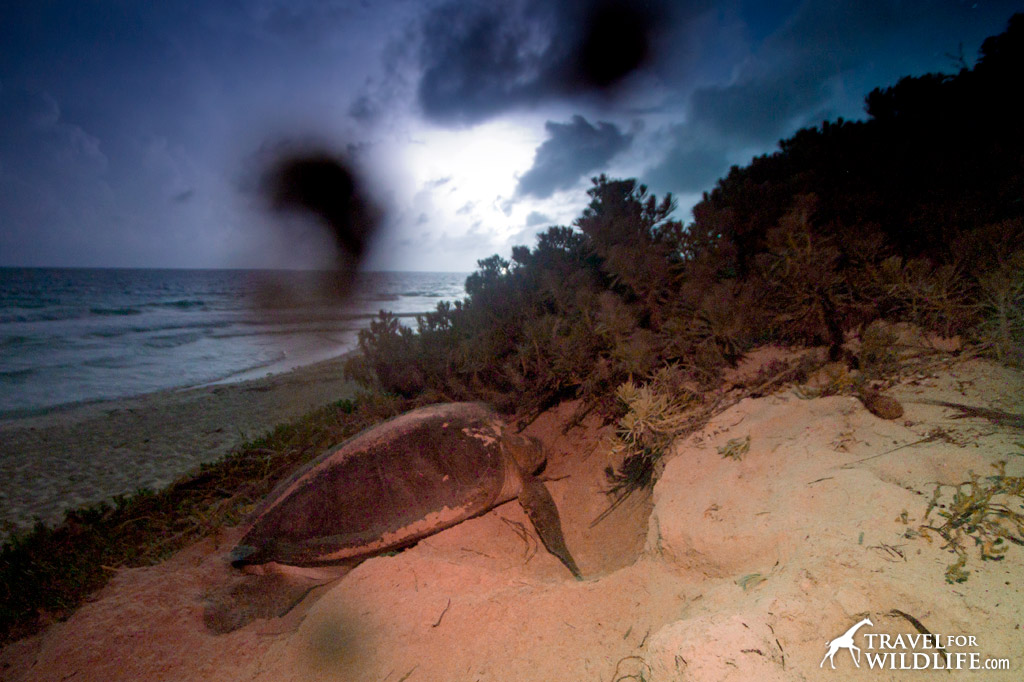In this outdoor photograph, a giant sea turtle is seen having emerged from the ocean and crawled onto a sandy hill at the edge of the beach, likely preparing to lay its eggs. The scene, taken during the impending nightfall, is shrouded in an eerie ambiance; the sky is a dark shade of blue filled with heavy, ominous clouds. A faint illumination hints at the presence of the sun or moon just beyond the frame. On the left side of the image, calm, gray water stretches out, bordered by dark green and brown bushes further adding to the night's shadowy vibe. The turtle, prominently positioned in the center of the image, is depicted with a brown shell and tan underbelly, its rear facing the camera as it digs into the tan sand. Scattered sand granules blur parts of the upper photograph, adding texture and a sense of immediacy to the action. In the bottom right-hand corner, a white silhouette of a giraffe and the text "travelforwildlife.com" subtly watermark the image.